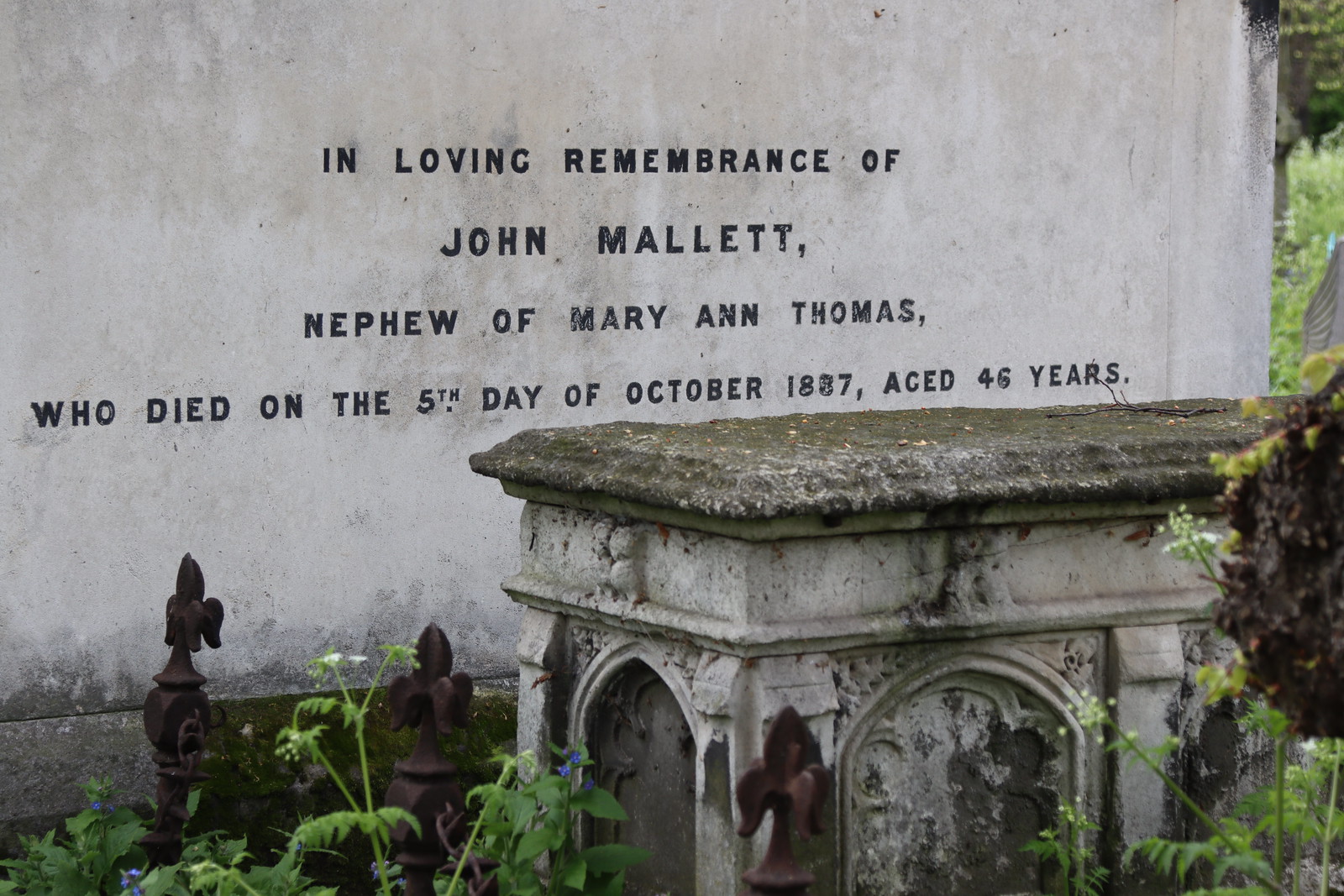The image is a digital photograph of a very old, weather-beaten cement tombstone, which serves as a memorial. The tombstone, surrounded by a rough, rusted iron fence, bears the inscription in black text: "In loving remembrance of John Mallett, nephew of Mary Ann Thomas, who died on the fifth day of October, 1887, aged 45 years." The cement structure is gray and appears worn with age, covered in moss and difficult to discern some of the finer details. The gravesite is enveloped by green grass, weeds, and bushes, adding to the sense of antiquity and abandonment. The memorial wall behind the tombstone also features the aforementioned inscription. The color palette of the image includes shades of green, black, gray, white, and blue, contributing to a somber and historic atmosphere.